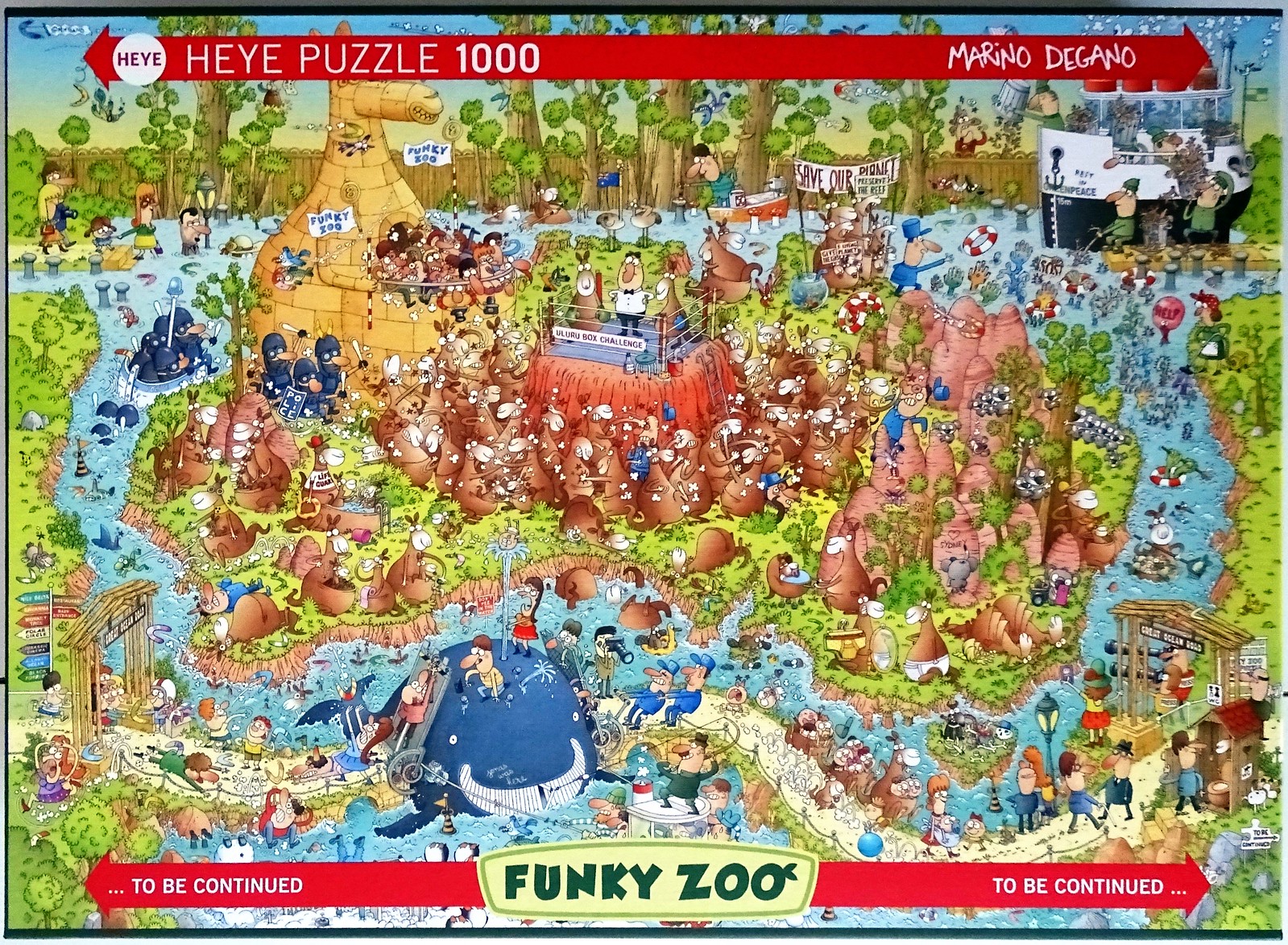The image is the cover of a search puzzle called "Funky Zoo" from the HEYE Puzzle 1000 series by Mariano Degano. The cover features a vibrant, cartoon-style illustration of an outdoor carnival set on an island surrounded by a river. The scene is bursting with activity and whimsical details. At the center of the island, an elevated boxing ring hosts a match between two anthropomorphic kangaroos, officiated by a referee, while photographers snap pictures nearby. The river teems with curious elements like a blue whale attempting to jump over a land bridge and various other aquatic doodads.

Prominent on the island to the left is a large, yellow stone structure resembling either a giraffe or a kangaroo. A bustling dock with a black-and-white cartoon boat fills the top right corner, and another dock appears at the top left. Among the greenery covering the island, there's a protest with signs to "Save Our Planet" and various humans and animals interacting, illustrating a zany coexistence. The puzzle's title, "Funky Zoo," is displayed at the bottom center in a playful green font, flanked by red arrows on either side that read "To Be Continued." The top of the box similarly features a red border with white lettering indicating it’s a HEYE Puzzle 1000 by Mariano Degano.